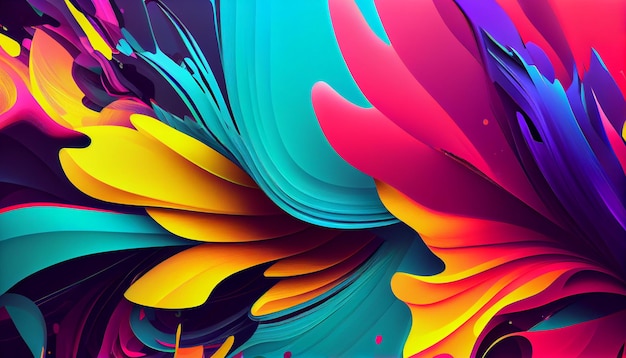This vibrant, rectangular digital painting, approximately five inches wide and three inches high, features a mesmerizing array of swirling colors and dynamic textures that evoke the sensation of movement. Beginning from the bottom right corner, the image bursts with swirls and fan-like strokes in vivid hues of red, pink, and yellow that resemble flowering petals and feather shapes. These colors gradually transition into a mix of gold, orange, and turquoise as they spread across the canvas.

Flowing upwards and towards the left, the composition transforms into broad strokes and strands of blue, teal, and aqua, which seamlessly blend with shades of purple. Darker tones of black and deep purple add depth, giving the impression of waves or dynamic currents moving gracefully to the left. Interspersed among these are streaks of gold with red veins and delicate petals-like designs that enhance the textural quality.

The abstract nature of this modern painting, with its vibrant color palette and intricate detail, creates an impression of perpetual motion and energy, as if waves and petals are continuously unfurling across the canvas toward the left.